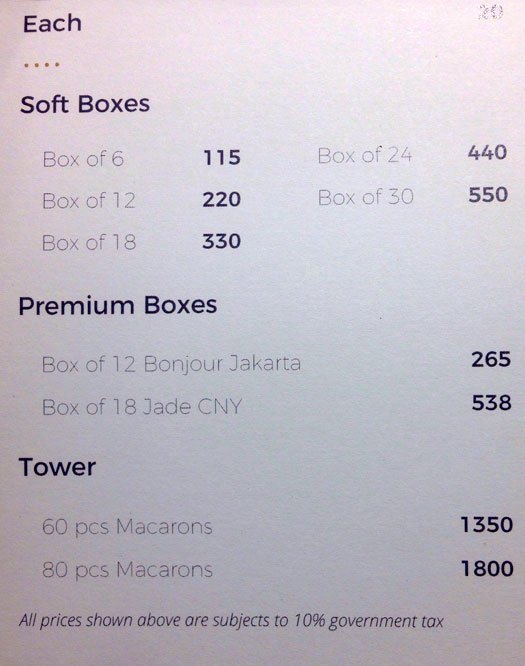The image is a detailed price list from a bakery, displayed on a light-colored paper. The layout is simple, with no pictures, and utilizes a straightforward font, with the titles and prices in bold while the rest of the text is in a lighter font. At the top, it features the word "Each" accompanied by four small yellow dots arranged in a vertical line. Below this are two main sections labeled "Soft Boxes" and "Premium Boxes." The prices for "Soft Boxes" are detailed as follows: Box of 6 for 115, Box of 12 for 220, Box of 18 for 330, Box of 24 for 440, and Box of 30 for 550. The "Premium Boxes" section includes: Box of 12 for 265 labeled as "Bonjour Jakarta" and Box of 18 for 538 labeled as "Jade CNY." Additionally, under the "Tower" section, the prices are listed as: 60 pieces of macarons for 1350, and 80 pieces of macarons for 1800. At the bottom, it notes that all prices are subject to a 10% government tax.